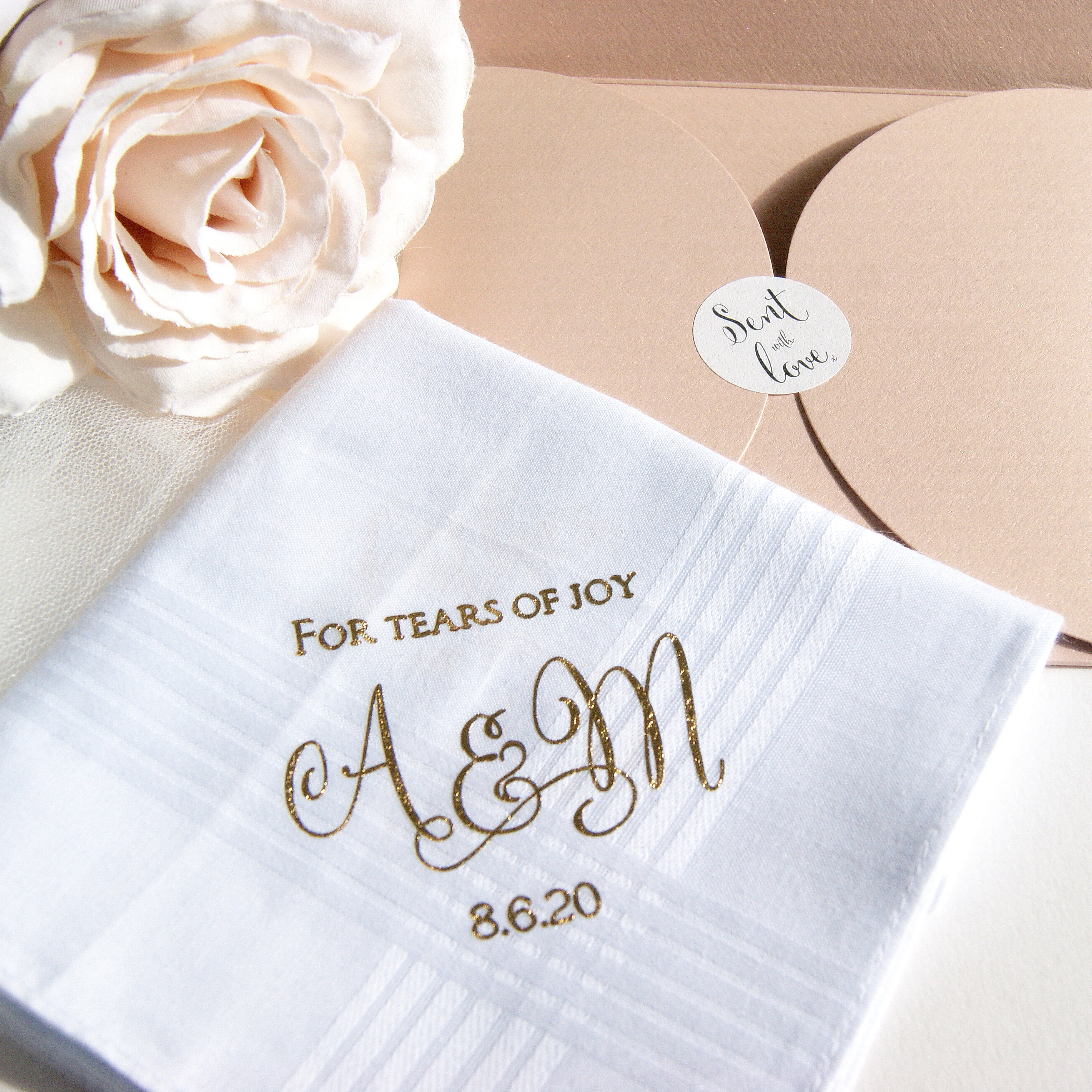This professionally shot image features a wedding gift set against a soft, pastel backdrop. At the center is a folded white linen handkerchief, displaying an intricate texture. Embossed in elegant gold letters on the handkerchief are the words "For Tears of Joy," alongside the initials "A&M" and the wedding date "8.6.20," indicating a special commission for a wedding on August 20th. To the top left, a pale pink rose with hints of peach hues complements the soft color palette. An off-white cardstock envelope, adorned with a gold-script "Sent With Love" sticker, sits at the top right, suggesting the handkerchief's luxurious packaging. This arrangement rests on a cream-colored linen tablecloth, creating a cohesive and romantic still life, perfect for an engraving or wedding gift advertisement.